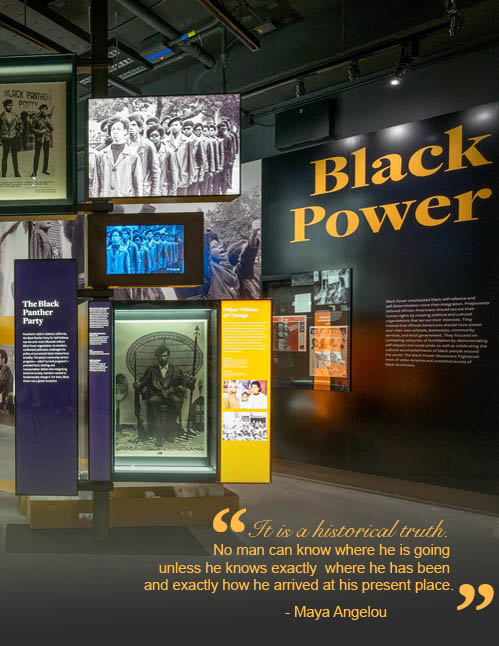The image is a detailed poster or exhibit entrance for a museum setup. Dominated by a vertical rectangular layout, the upper portion prominently displays the words "Black Power" in bold orange text. Below, the image features a thoughtful quote from Maya Angelou in both cursive and print that states, "It is historical truth. No man can know where he is going unless he knows exactly where he has been and exactly how he arrived at the present place," flanked by large quotation marks. 

The scene within the image suggests the entrance to an exhibit focused on historical content, possibly about the Black Panther Party, given the mention against a purple-colored caption on the left. The exhibit includes various displays: an elephant, several informational panels with text, and a series of television monitors attached to a metal pole, all under an unfinished ceiling that reveals pipes and wires, contributing to a warehouse aesthetic. Banners of different colors, such as purple and yellow with white text, flank the displays, enhancing the exhibit's informative nature. Photographic imagery of African-American individuals is also present, underscoring the exhibit's historical emphasis.